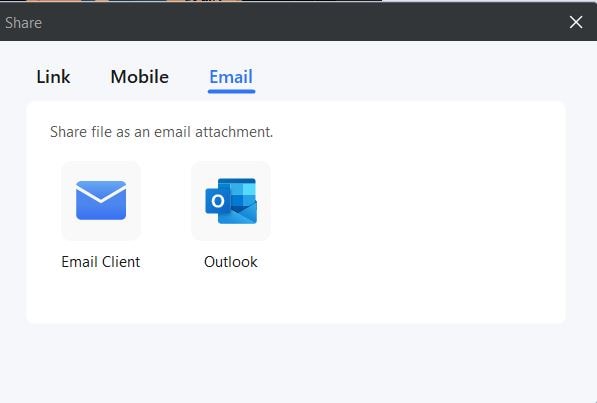This is a screenshot of an application interface featuring a black bar at the top with a white 'X' icon in the right corner, which likely serves as a close button. Below the black bar, there are three navigational tabs: "Link," "Mobile," and "Email," with "Email" highlighted in blue and underlined by a blue line, indicating it is the currently selected tab. Underneath these tabs, the text "Share file as an attachment" is displayed in a grey font, followed by "Email Client" written in black. There is an envelope graphic icon next to the word "Outlook," which is written in black font and accompanied by the Outlook logo.